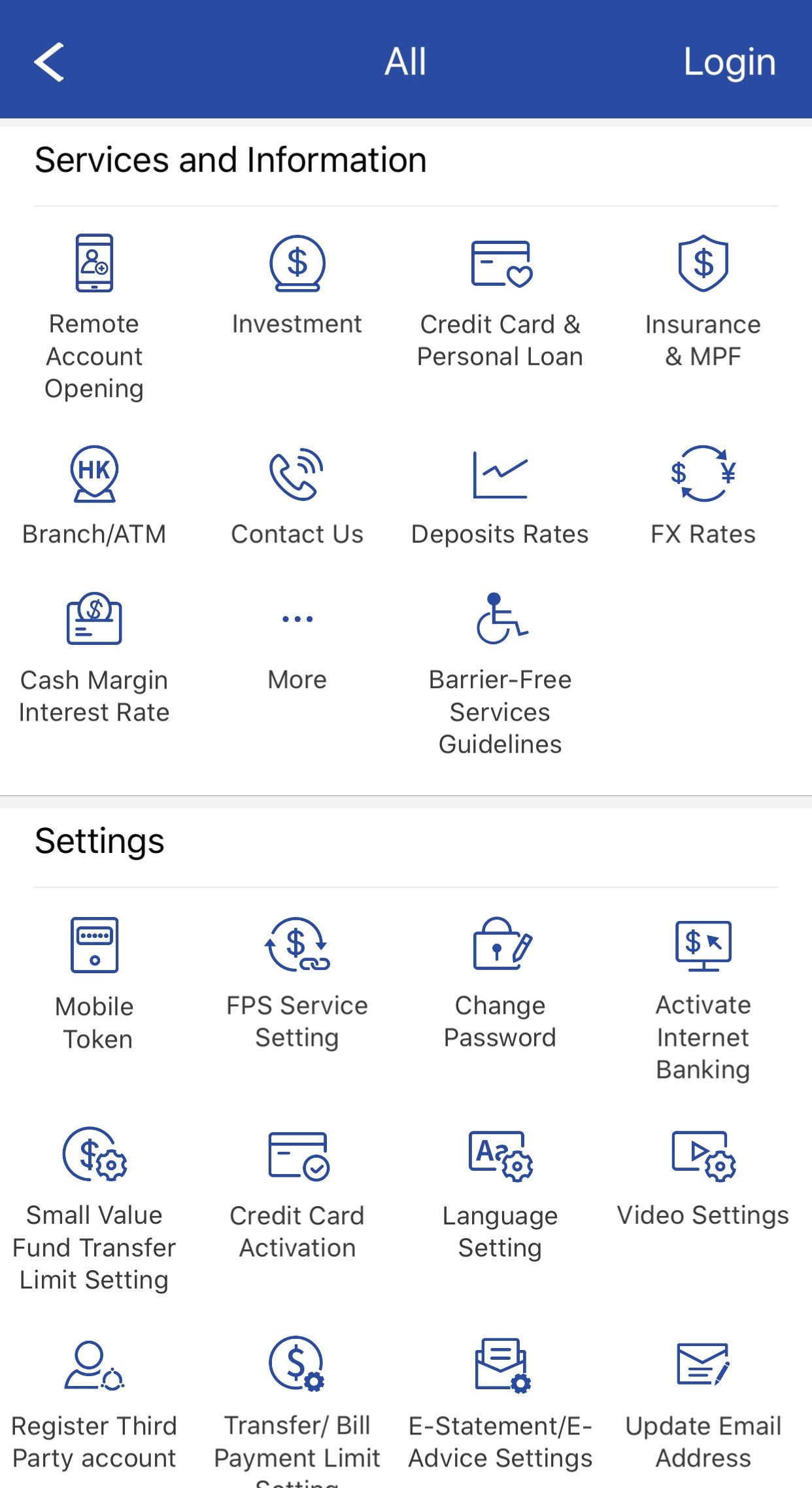The image depicts a cell phone screen with a user interface divided into two main sections against a predominantly white background. The screen is a tall rectangle primarily organized into an upper pane labeled "Services and Information" and a lower pane labeled "Settings."

At the very top of the screen, a blue band stretches horizontally. Within this band, on the left side, there is a left-facing caret icon. Centered in white text, the word "All" is displayed, and on the right side, also in white text, is the word "Login."

The "Services and Information" pane follows, clearly demarcated in dark type. This pane contains eleven icons organized in a grid of three rows. Each row can accommodate four icons, but the last spot in the final row is intentionally left blank. The first row features the following icons from left to right: 
1. Remote Account Opening
2. Investment
3. Credit Card and Personal Loan
4. Insurance and MPF

The second row contains:
1. Branch/ATM
2. Contact Us
3. Deposits Rates
4. FX Rates

In the third row, the icons and labels are:
1. Cash Margin Interest Rate
2. More
3. Barrier-free Service Guidelines
4. (This spot is blank)

Below that is the "Settings" pane, set off in darker type. This pane is also divided into a grid format, with sixteen icons distributed evenly across three rows. Each row consists of four icons. The first row includes:

1. Mobile Token
2. FPS Service Setting
3. Change Password
4. Activate Internet Banking

The second row displays:
1. Small Value Fund Transfer Limit Setting
2. Credit Card Activation
3. Language Setting
4. Video Settings

The third and final row features:
1. Register Third Party Account
2. Transfer/Bill Payment Limit
3. E-Statement
4. E-Advice Settings
5. Update Email Address